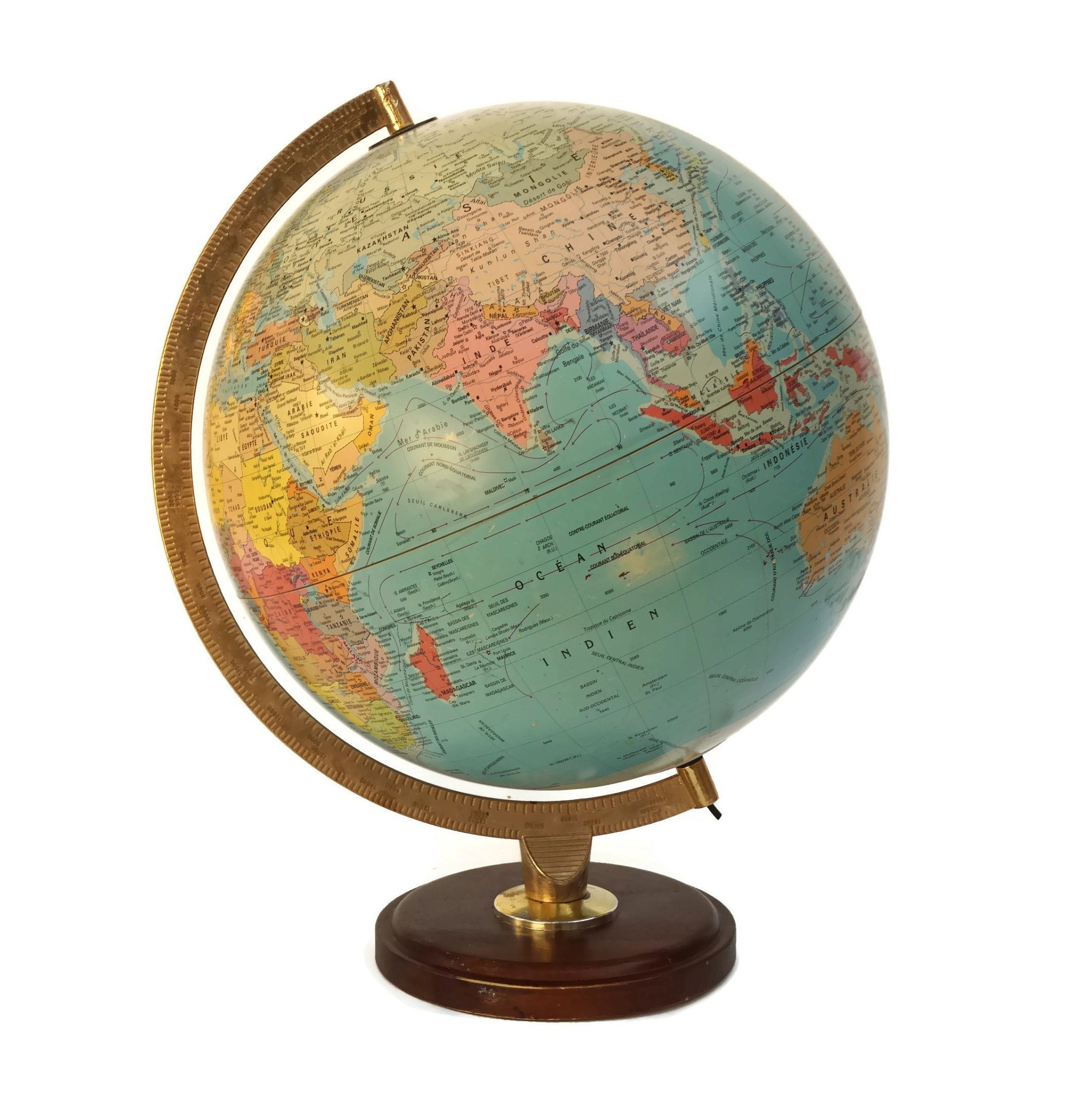In the image, there is a classic globe mounted on a tripod with a brass half-ring meridian framing it. The globe vividly displays an intricate section of the Earth, featuring the Indian Ocean prominently in the center. To the right, Australia is depicted in a brown shade. Adjacent to the left, the right side of Africa is visible alongside the Middle East, showcasing a multicolored terrain. Above them, India is rendered in a pinkish hue, while China exhibits a slightly lighter shade of pink. Further north, Russia stretches out with its vast expanse, and Japan stands out near the globe's edge in a striking red color. The ocean waters are rendered in blue, providing a stark contrast to the distinctive land colors. The globe is supported by a sturdy tripod, which culminates in a small, round wooden base, giving the entire setup an elegant and classical appearance.